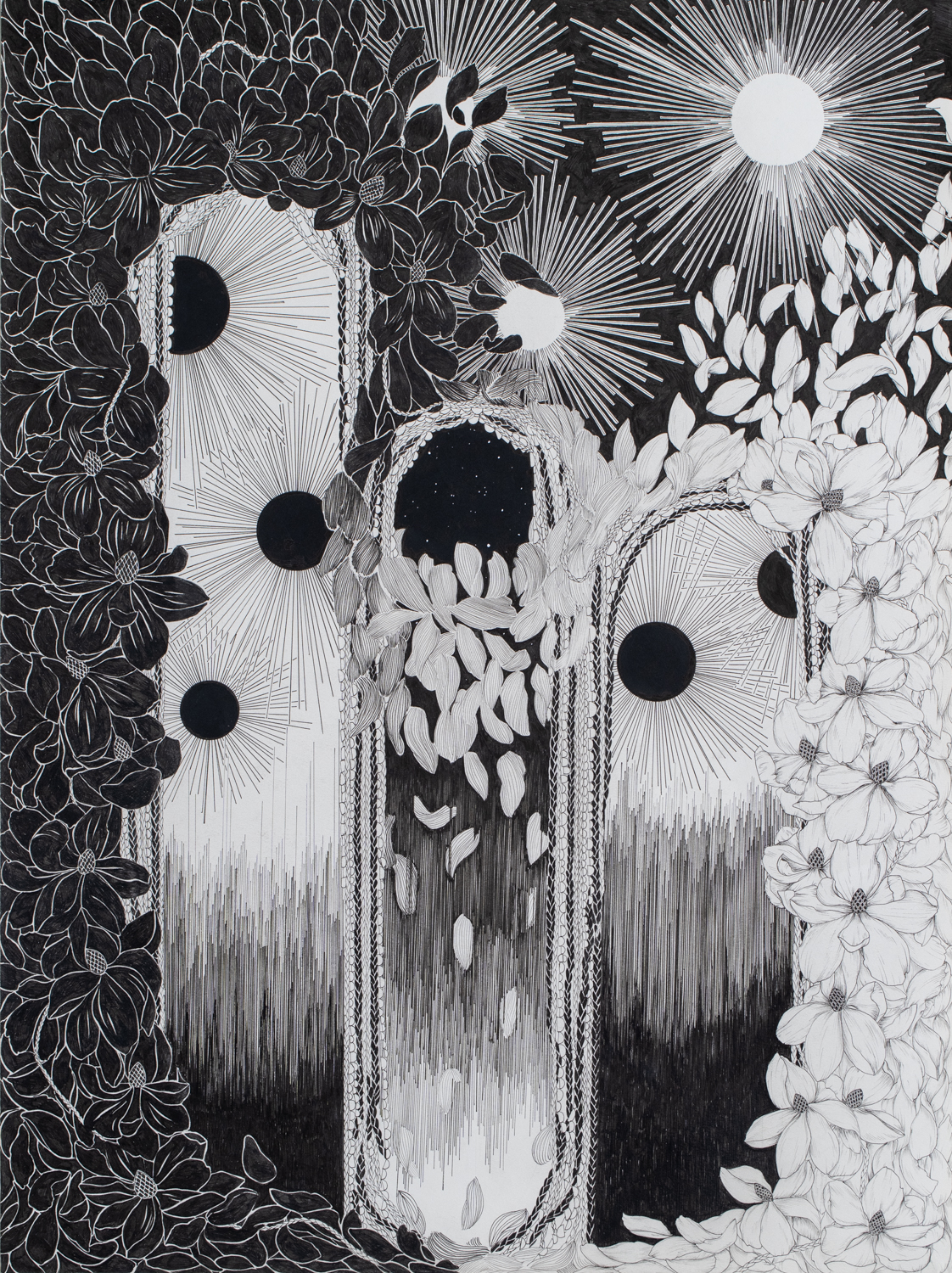A rectangular sketch, approximately six inches tall by four inches wide, rendered in deep charcoal or pencil, showcases a striking contrast between void-black and varied whites. The left side of the image is dominated by intensely black flowers, while the right side features white blooms, creating a yin-yang effect. In the background, multiple suns with white centers and thin beams radiate from the upper right corner, set against a dark backdrop. Dark flowers and leaves arch from the center, forming a canopy around the suns, which also appear in black variants with black beams. The center of the image contains three oval, mirror-like forms of varying heights, draped in flowers and seemingly reflecting the suns. Surrounding these mirrors are black leaves and white petals, resembling a night sky above and cascading white petals below. The detailed, starburst-like blossoms with thin petals add to the ethereal and surreal quality of the artwork.